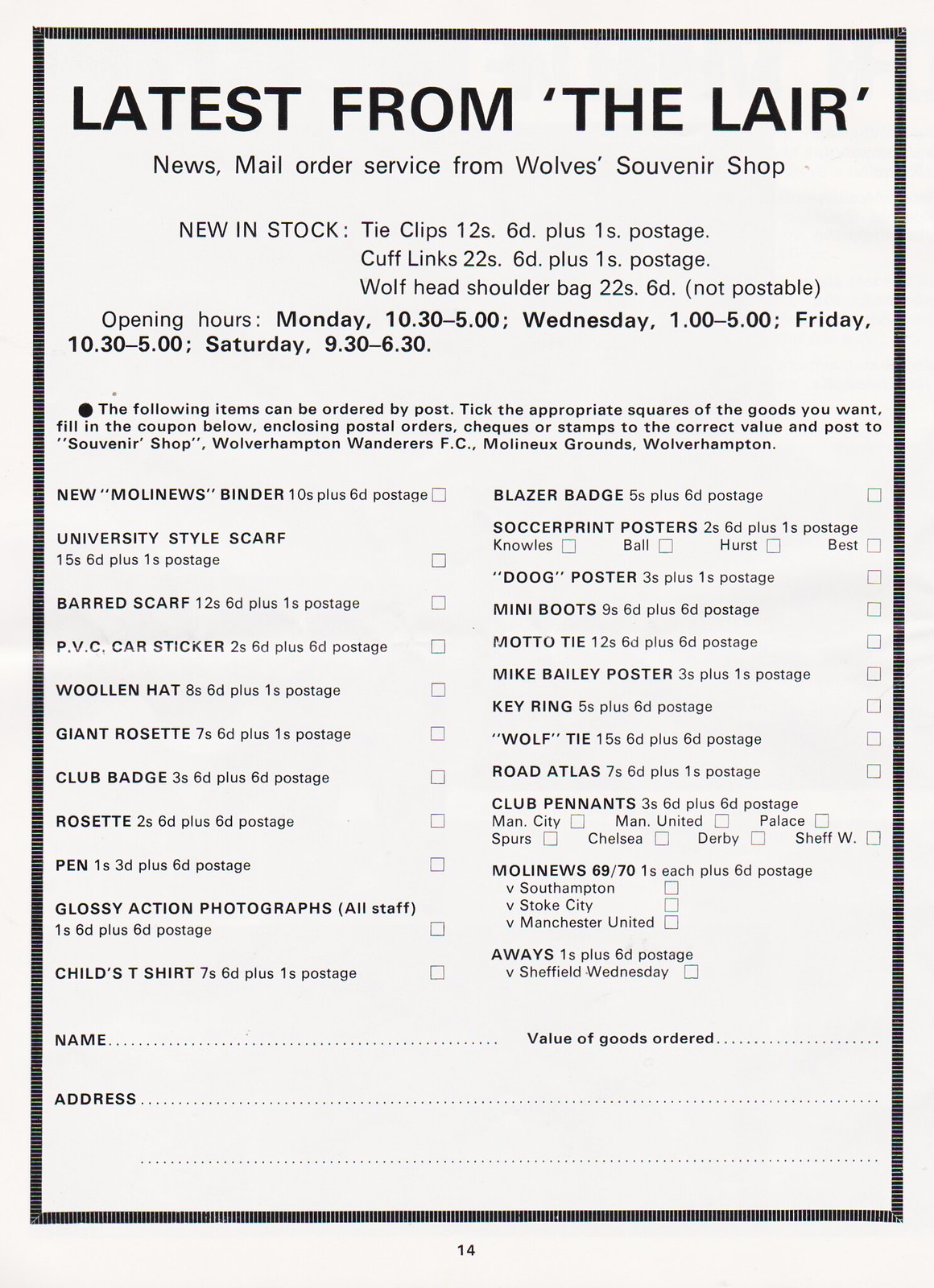The image depicts an order form from a Wolves Souvenir Shop, likely torn from a magazine, set against a light blue background. At the top, the heading reads, "Latest from the Lair News - Mail Order Service from Wolves Souvenir Shop." The text highlights new in-stock items such as tie clips (12s 60 plus 1s postage), cufflinks (22s 60 plus 1s postage), and a wolf head shoulder bag (22s 60, specified as not postable). Opening hours are listed as Monday 10:30 to 5, Wednesday 1 to 5, Friday 10:30 to 5, and Saturday 9:30 to 6:30. 

The form is organized into two columns with several items available for order, each accompanied by a checkbox for selection:
- New Molyneux Binder (10s plus 60 postage)
- University Style Scarf (15s 60 plus 1s postage)
- Banded Scarf (12s 60 plus 1s postage)
- PVC Car Sticker (2s 60 plus 60 postage)
- Woolen Hat (8s 60 plus 1s postage)
- Giant Rosette (7s 60 plus 1s postage)
- Club Badge (3s 60 plus 60 postage)
- Standard Rosette (2s 60 plus 60 postage)
- Pen (1s 3d plus 60 postage)
- Classy Action Photographs (1s 60 plus 60 postage)
- Child’s T-Shirts (7s 60 plus 1s postage)
- Blazer Badge (5s plus 60 postage)
- Soccer Print Posters (2s 60 plus 1s postage)
- Posters of players like Knowles, Ball, Hearst, and Best
- Duke Poster (3s plus 1s postage)
- Mini Boots (9s 60 plus 60 postage)
- Motto Tie (12s 60 plus 60 postage)
- Mike Bailey Poster (3s plus 1s postage)
- Keyring (5s plus 60 postage)
- Wolf Tie (15s 60 plus 60 postage)
- Road Atlas (7s 60 plus 1s postage)
- Club Pennants with team names like Man City, Man United, Palace, Spurs, Chelsea, Derby, Sheffield Wednesday
- Molyneux 69-71 editions (each 60 postage)
- Specific match items for Southampton, Stoke City, Manchester United, Sheffield Wednesday
- "Aways" (1s plus 60 postage)

Below the listings, there is a space to fill out the customer’s name, address, and value of the goods ordered. Instructions for ordering by post are provided, indicating that customers should tick the appropriate boxes, fill in the coupon, and send postal orders, checks, or stamps to the correct address at the souvenir shop located on the Molyneux grounds in Wolverhampton.